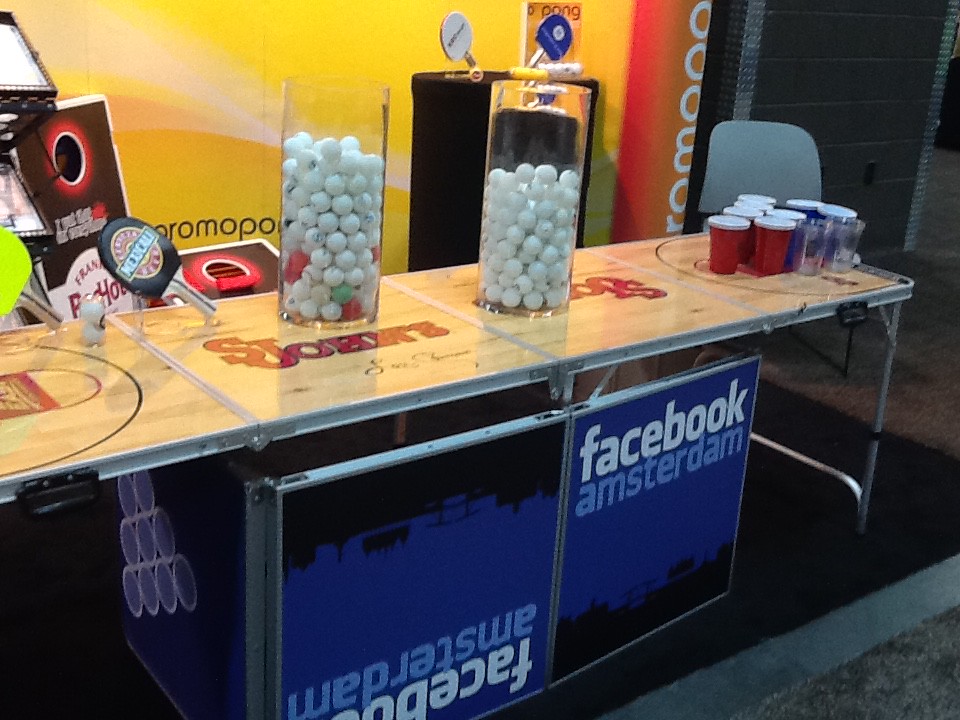The image features a wooden ping pong table with metal legs, likely repurposed for a drinking game setup similar to beer pong. At one end of the table, several red and blue solo cups are arranged in triangular formations, accompanied by clear cups. Two large clear containers filled with an estimated 30 to 40 ping pong balls each are prominently situated at the center. Additionally, two ping pong paddles lie on the left side of the table. The table is labeled "St. John's" on its surface and bears signs that read "Facebook Amsterdam" both right-side-up and upside down. In the background, a yellow banner is visible, along with several display cases containing ping pong paddles and tennis rackets. Underneath the table, there's a cluster of solo cups seemingly connected or glued together, enhancing the setup's impression of being intended for a beer pong game or a similar activity.